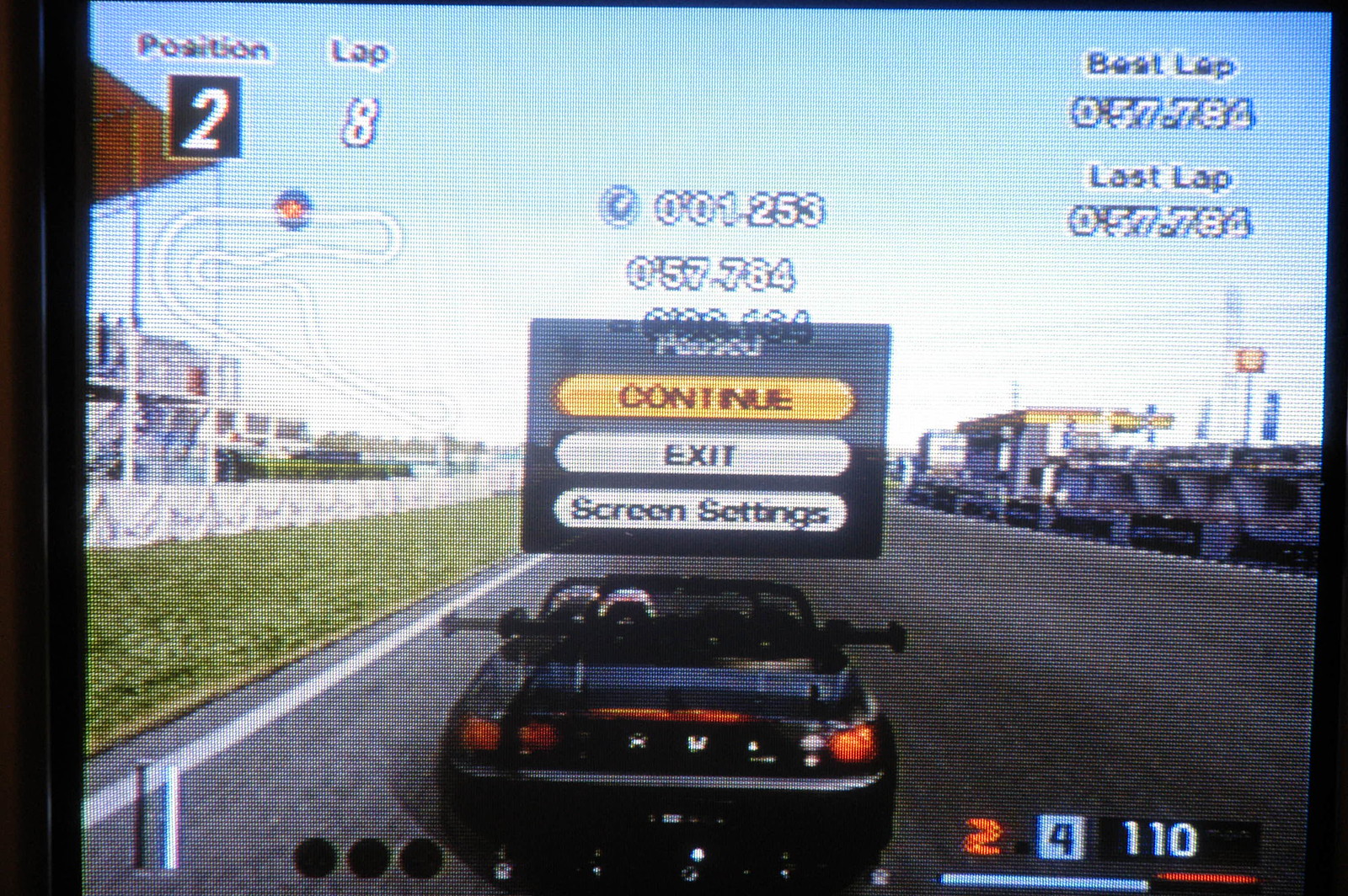The image features a screenshot of a classic racing video game, likely from the early 2010s, captured using a phone, evident from the quality. The scene is paused, displaying a menu with "Continue," "Exit," and "Screen Settings" options at the center. The game showcases a sleek, black sports car, with essential racing data populating the screen. On the top right, there is a display indicating the lap number and the last lap time. The bottom right corner hosts the car's speedometer and current gear information. The top left of the screen features a lap counter, the player's race position, and a mini-map of the racetrack, providing a comprehensive overview of the player's progress in the race.